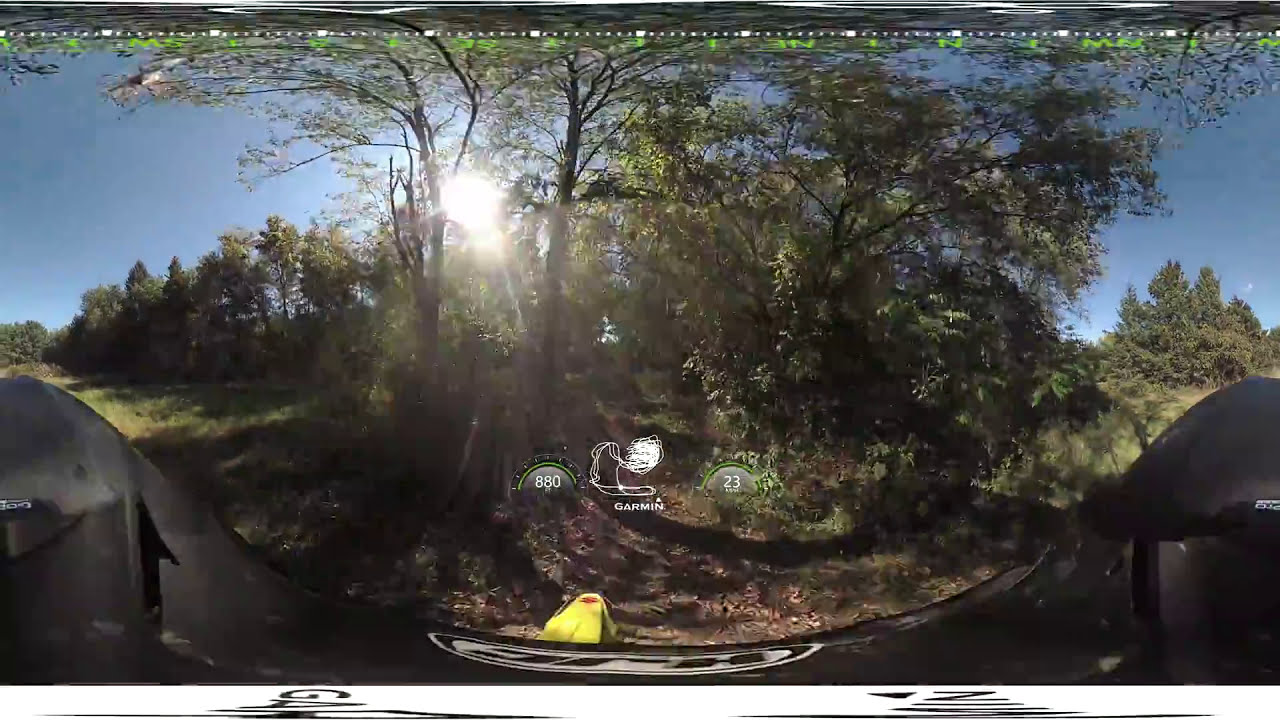The grainy image, likely captured by a GoPro or dash cam mounted on an ATV, depicts a rugged forest terrain on a dirt path covered with wood chips. The path is flanked by dense, leafy trees and bushy fields, suggesting a summertime setting, although some bare branches hint at the late summer stages. The wide-angle shot, possibly from a fisheye lens, creates noticeable distortion, particularly around the edges. A Garmin watermark with various metrics is prominently displayed in the center, along with some yellow logo, and additional overlay icons including the numbers 800 and 880. The clear blue sky with the sun peeking through the foliage adds to the scenic atmosphere, while visual distortions and black areas appear on the left and right edges, contributing to the unique aesthetic of the photograph. A windshield can be seen on either side of the dashboard, reinforcing the movement through this vibrant, dynamic forest landscape.